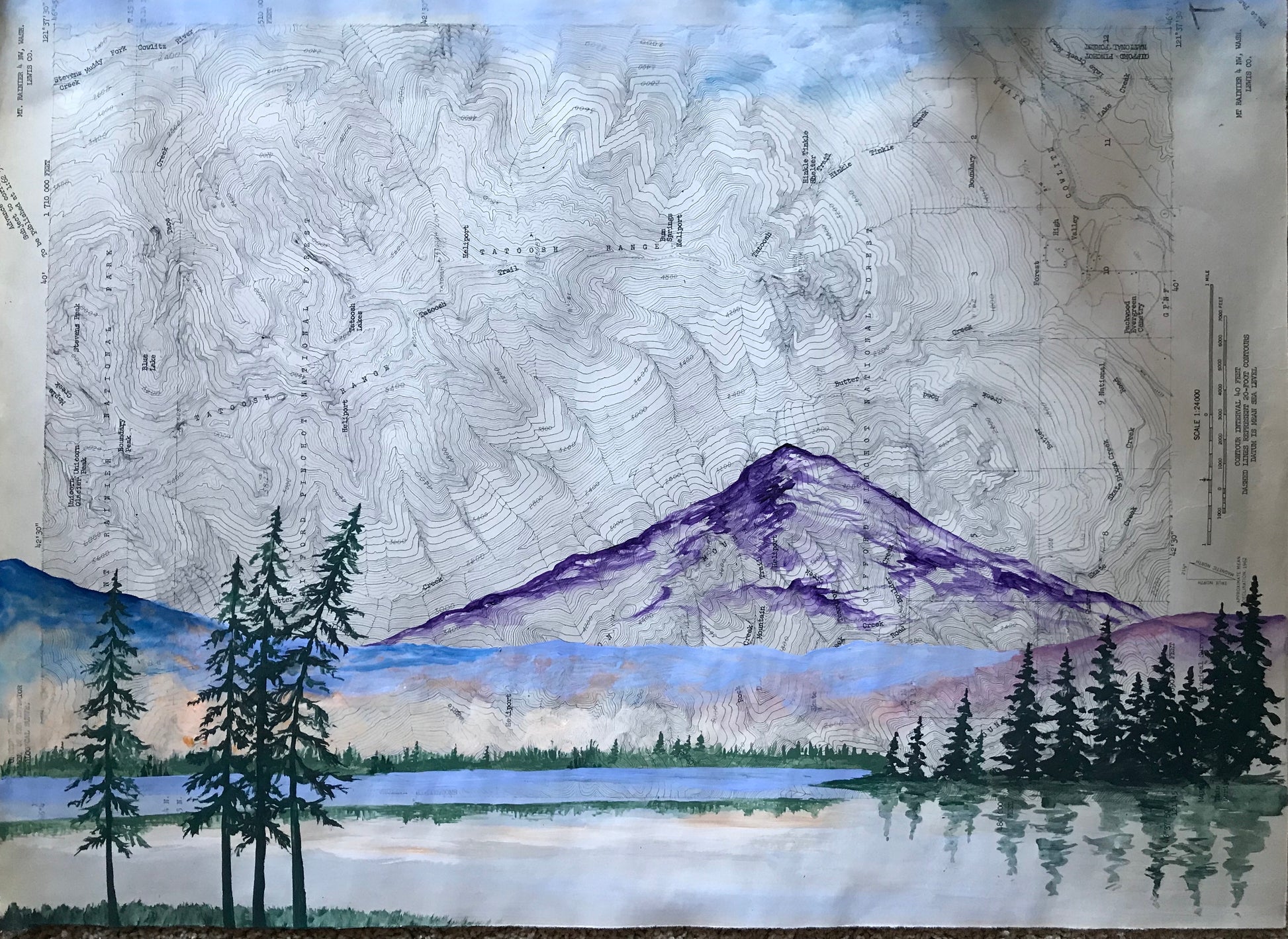The artwork depicts a striking mountain scenery crafted with meticulous clay art. Dominating the background, a topographical map showcases the intricate waves, hills, and valleys of a mountain pass in primarily black and white, with hints of light sky blue at the top. Centrally, a majestic mountain stands out in rich purples and whites, with another, more gradual, bluish-purple mountain nested below it. The foreground features a tranquil lake, reflecting the scenery around it, including small patches of dark green pine trees on the left side and taller pines on the right. Four tall green trees mark the left front corner. The area surrounding the lake transitions from clear water in the front to patches of white and green grass. The entire scene is unified by lines indicating varying elevations, subtly embedded into the background to represent the mountain's topographical details.